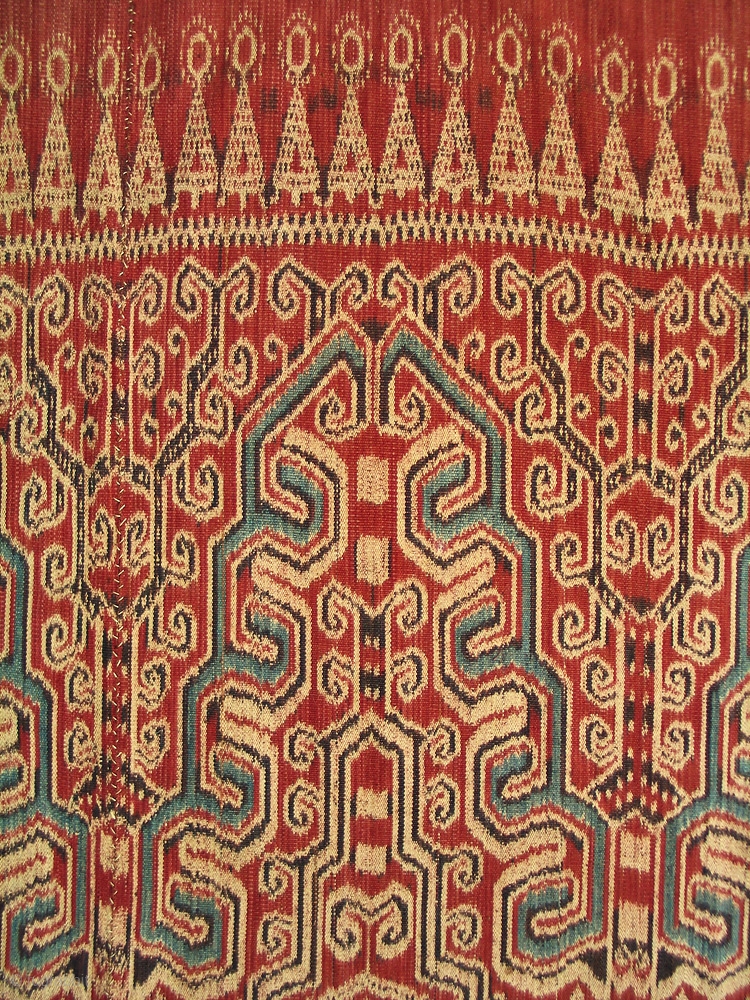The image features an intricate woven cloth, identified as an Ikat ritual cloth, known as a Pua, originating from the Kalimantan-Sarabas border region of Indonesia, dating between the 1920s to 1940s. This ceremonial hanging is made from cotton dyed with natural colors, and showcases a rich tapestry of burnt red, dark teal, beige, and black hues. The design is a mirrored pattern that converges into a pointed central motif, adorned with triangular shapes resembling teepees or a-shapes with circular openings at their apex. Beneath these triangles lies a complex, sophisticated design that includes curled scrollwork and vine-like motifs, intertwined in black, gray, green, and red. Central to the pattern is a prominent blue element, outlined in black and white, which gives the piece a balanced yet intricate aesthetic. The entire cloth exudes not only beauty but also cultural significance, reflective of its origins and the artisanal skill of the weavers from the Sarabas border region.